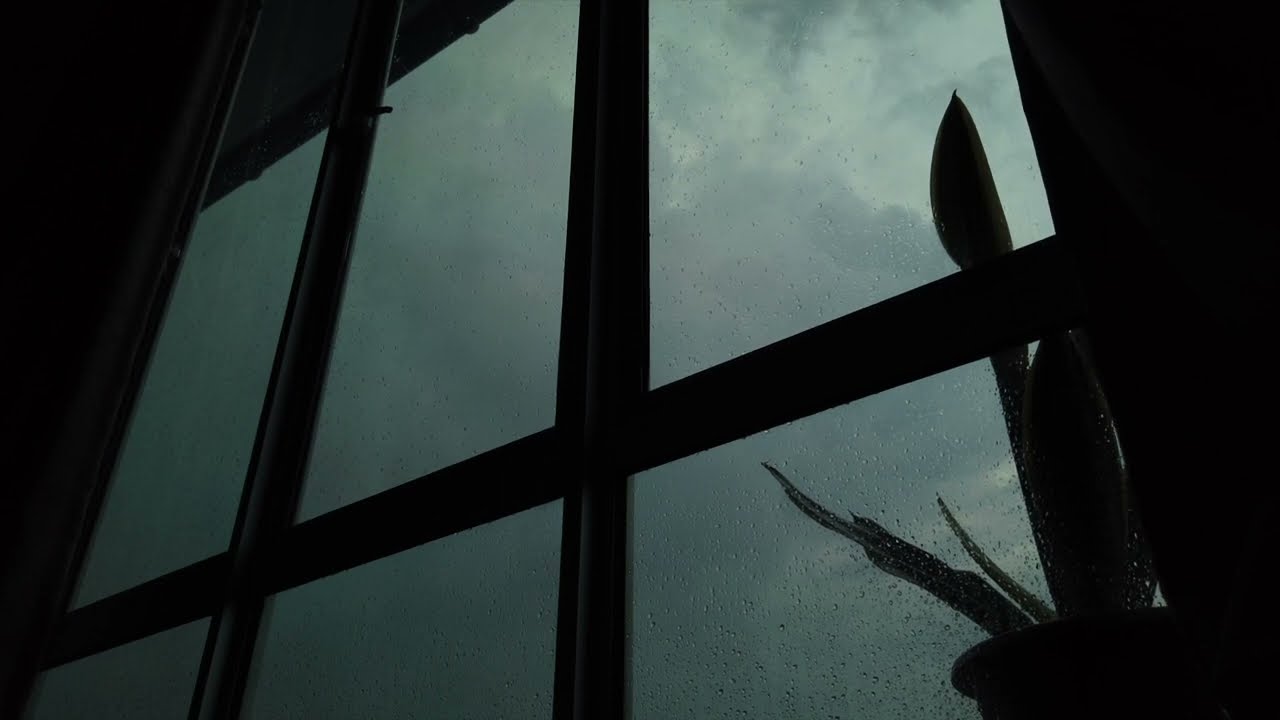The photograph captures the view from inside a dark building, looking out through a large window with six rectangular panes divided by black bars. The perspective is angled upward towards the left, focusing on a stormy sky dominated by dark gray rain clouds with patches of white. Water droplets cling to the panes, particularly concentrated in the bottom right section. A silhouette of a potted plant, possibly a fern with large leaves, is seen in the bottom right corner of the window, with one branch stretching straight up and another extending towards the upper left. Shadows cast over the scene make the details harder to discern, and remnants of the building's eaves can be glimpsed in the upper left part outside the window.